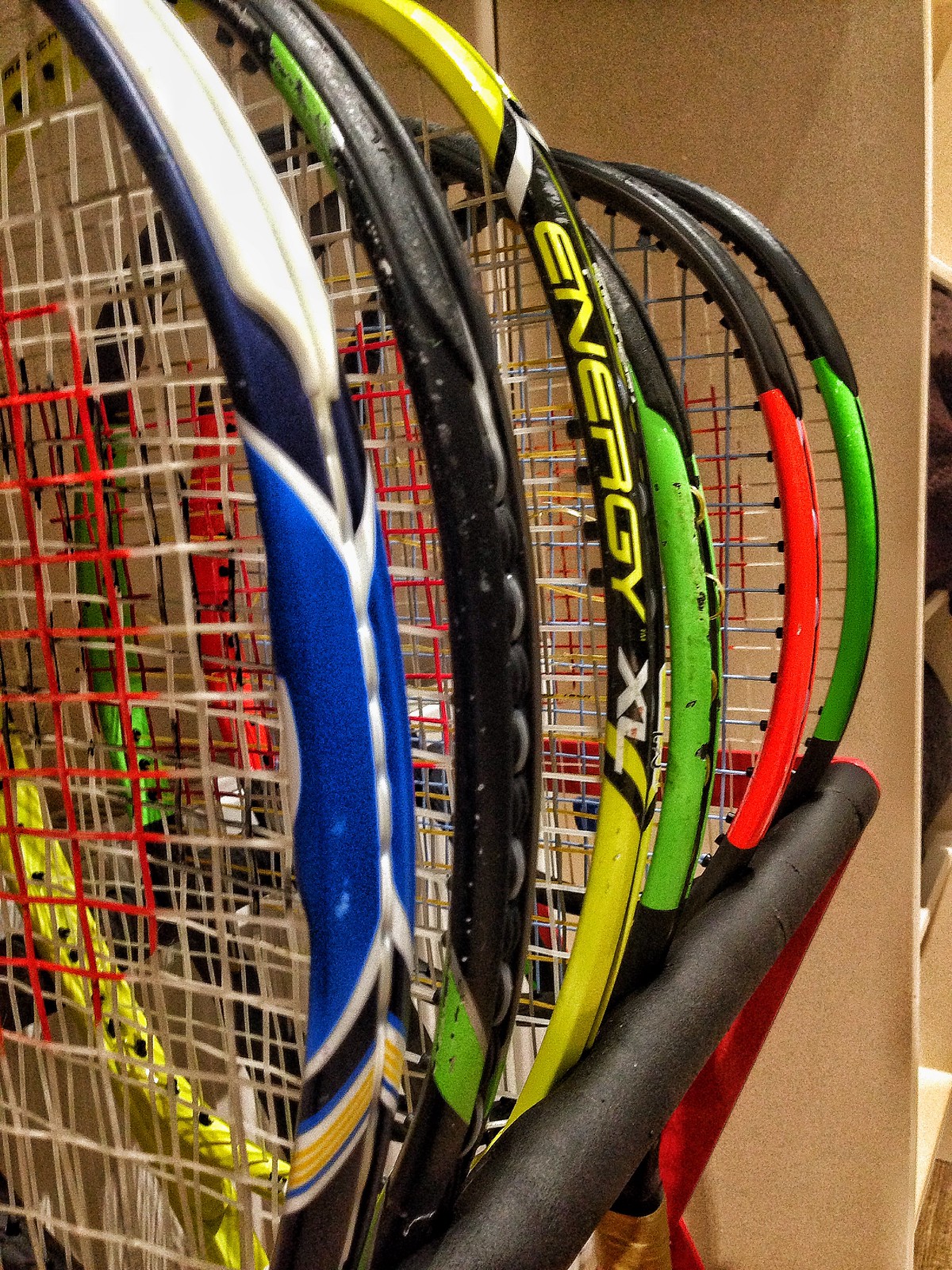This detailed close-up photograph captures a red metal tennis racket rack, cushioned with black foam padding, showcasing six tennis rackets neatly arranged side by side. The photograph zeroes in on the widest part of the rack, with only the heads of the rackets visible. The racket closest to the camera features a striking frame in blue, black, white, and yellow, and prominently displays a red logo on its strings. Beside it, the next racket has a sleek black frame accentuated with lime green stripes. Moving along, the third racket also in black, features the words "Energy XL" with "ENERGY" written in yellow on a black background and "XL" in white letters. Another racket displays a wide lime green stripe on a black frame, while the next one has a broad red stripe against a black background. The last racket in the arrangement sports a wide stripe in green. All rackets are supported by a red metal frame with a black foam bar, efficiently holding them in place like a specialized bookcase.